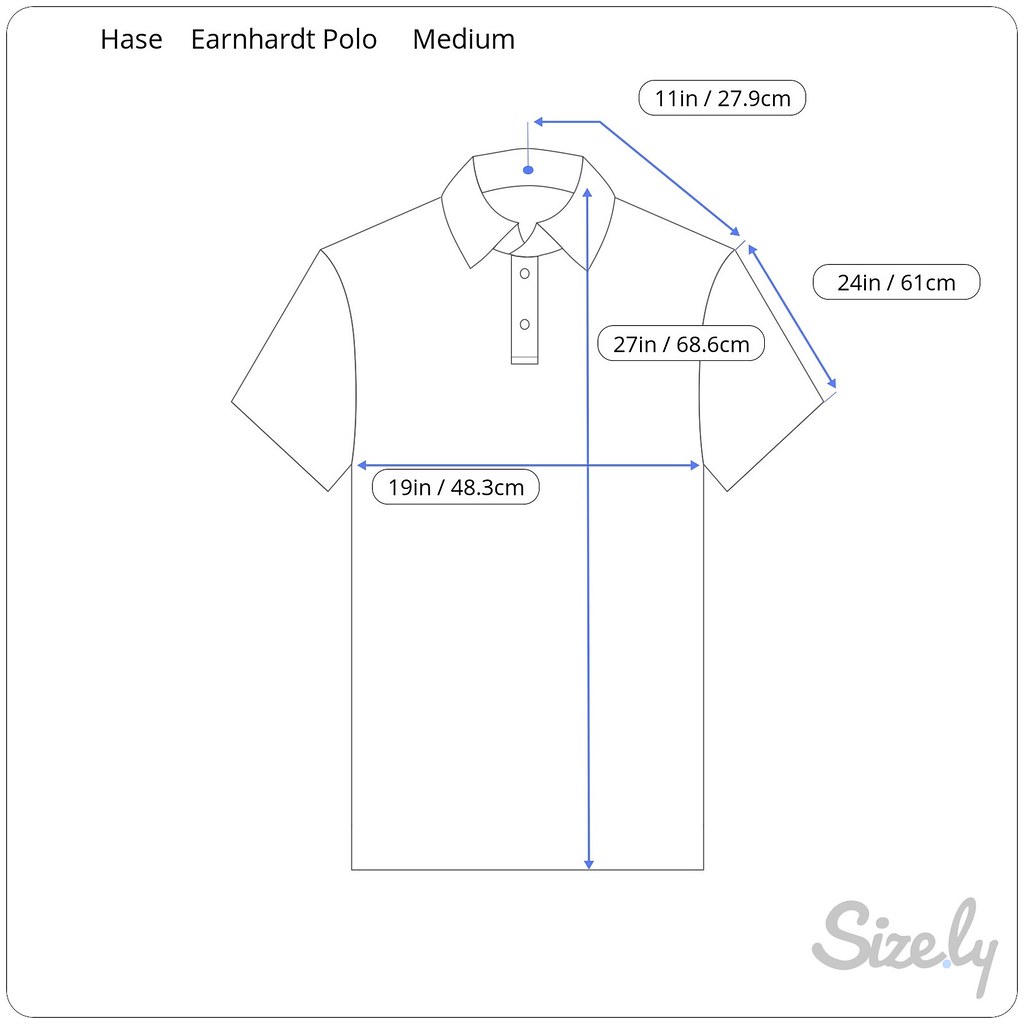This detailed schematic drawing depicts a short-sleeved, button-down shirt with precise measurements, resembling an architect's blueprint. Set against an all-white background and encased in a thin black border, the shirt's dimensions are marked with blue measurement lines featuring arrows at both ends. The shirt, centrally positioned, has a collar with three buttons and rounded corners making the image nearly square. Above the diagram, in black letters, it states: "Hace, Earnhardt, Polo, Medium." The measurements are as follows: a vertical line from the collar to the bottom measures 27 inches (68.6 cm), a horizontal line across the chest measures 19 inches (48.3 cm), the sleeve length from the shoulder is 24 inches (61 cm), and from the top of the sleeve to the center of the collar is 11 inches (27.9 cm). In the bottom right corner, a light gray logo reads "Sizely." The primary colors used are black, white, blue, and gray, contributing to the documentary-like aesthetic of this printout.